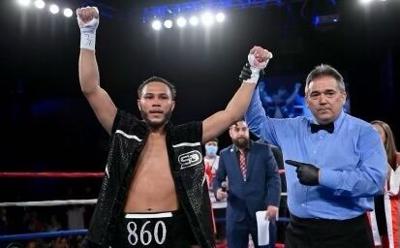In the dimly lit setting of what appears to be a boxing championship, the arena's dark background contrasts sharply with bright stage lights hanging in rows from the rigging above. Red, blue, and yellow boxing ropes encircle the ring, partially visible behind a crowd of blurred spectators. Central to the image are five distinct figures. In the front, a victorious boxer stands with his wrists wrapped in white tape, both arms raised. He wears a black and white vest, open in the front to reveal his torso, and black shorts emblazoned with "860" in large white digits.

The referee, positioned next to him, proudly holds up the boxer’s left arm. Dressed in a blue long-sleeve shirt, black bow tie, black pants, and black gloves, he points towards the winner with his other hand. Just behind them, a man donning a blue suit and red-and-white checkered tie holds some papers, his dark hair and beard visible. Further back, partially obscured, a man in a white and red shirt with a medical face mask and a possible bandana stands, alongside a woman hidden behind the referee, identifiable by her long light brown hair and red and white attire resembling a boxing robe. The vivid lights above cast a stark glow on the victorious moment, encapsulating the energy and spectacle of the event.